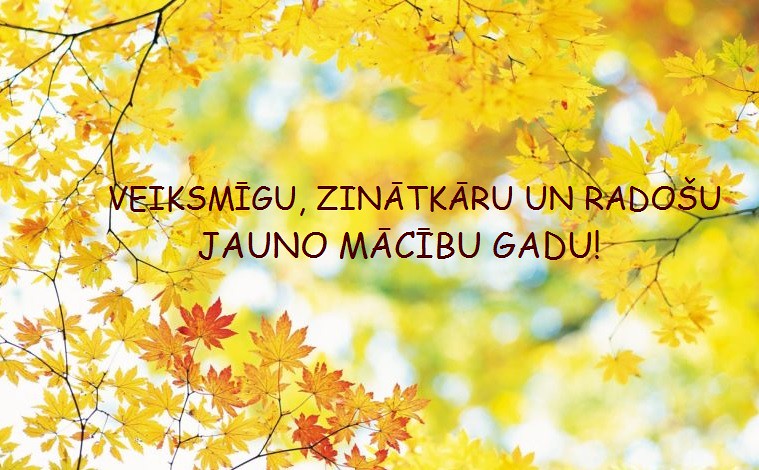The image is a horizontally aligned rectangular graphic that encapsulates the essence of an autumn day. It features partial branches adorned with vibrant orange, yellow, and red seven-pointed leaves enveloping the border. The center of the image is deliberately blurred, offering hints of a bright, outdoor scene with shades of yellow, green, white, and blue, likely showcasing the sky peeking through the foliage. Centered in the image are two lines of text in a foreign language, composed of approximately seven letters per line, resembling an inspirational quote or message, written in black letters. This striking visual juxtaposes the sharp, colorful details of the autumn leaves against the subtly blurred background, capturing a fleeting moment of natural beauty.